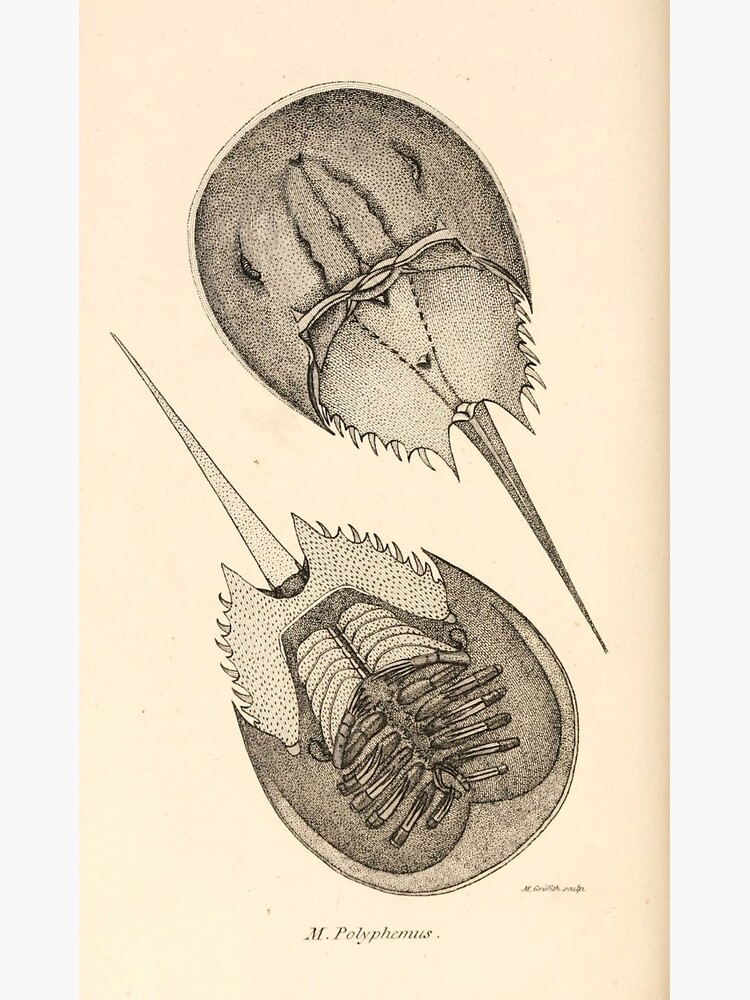The image is a detailed black and white illustration of a horseshoe crab, drawn on old, yellowing paper. The illustration presents two perspectives: a top view and an underside view. The horseshoe crab is depicted with a rounded, almost egg-shaped body, tapering into a long, sharply pointed tail. The top view reveals the creature's segmented carapace with its characteristic three lines running through the forehead area and small slits indicating its eyes. On both the top and underside, there are multiple spikes along the sides of the body.

The underside view shows the crab's numerous appendages, detailing at least six legs on each side, each ending in claw-like pinchers. The tail, also visible from this angle, is elongated and pointed, with the entire illustration marked by intricate black dots adding texture and detail to the creature's body. 

The background of the image is a light tan or off-white color, enhancing the contrast with the grayscale illustration. The bottom of the image is labeled with "M. Polyphemus," and additional writing on the right side appears to credit the artist as "M. Griffith," though some parts of the text are unclear. The horseshoe crab, though described as rather plain and unappealing, is meticulously rendered to highlight both its form and function.